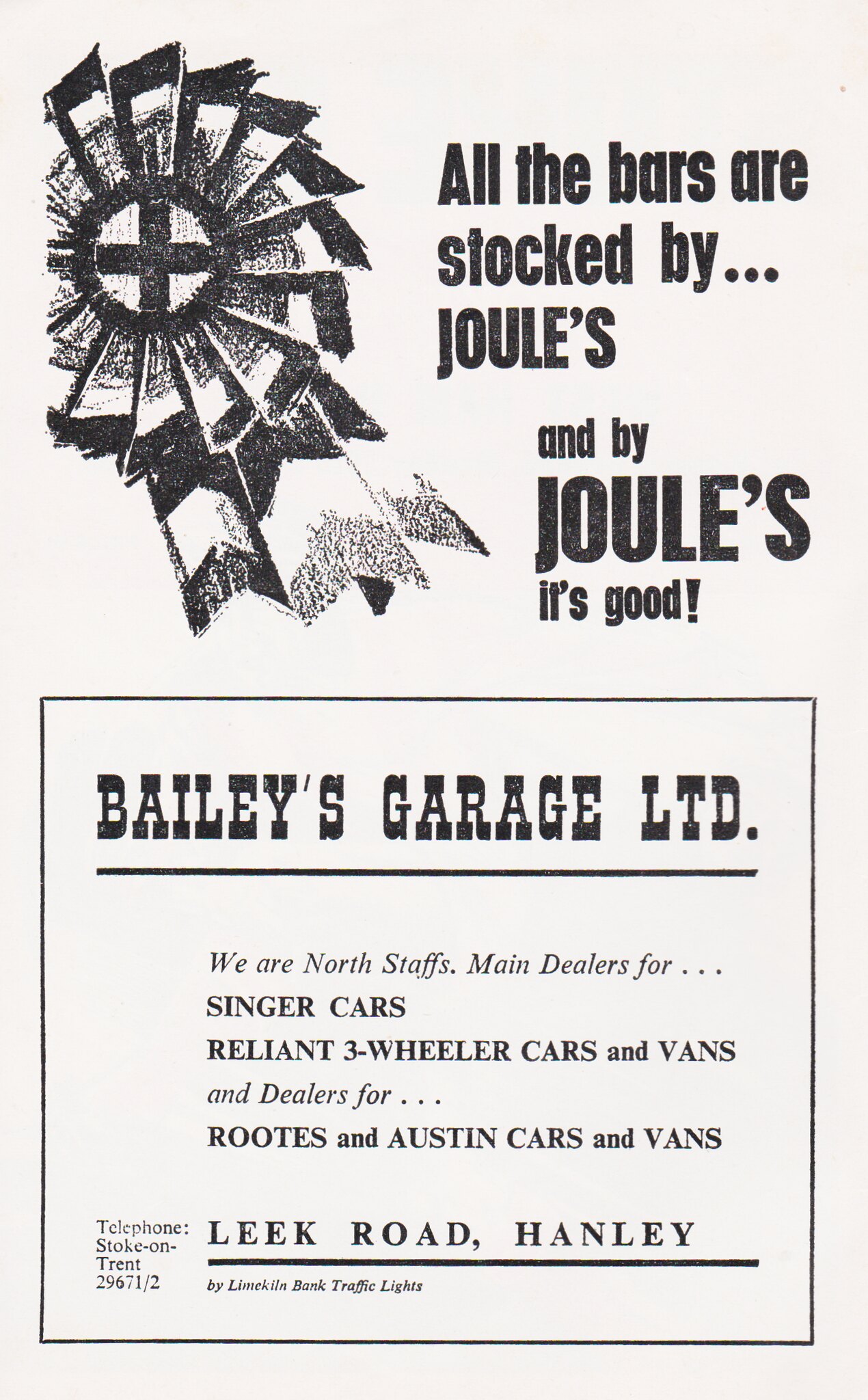This image appears to be a black-and-white scan of an old advertisement from a magazine or pamphlet. The upper half features a drawing of a ribbon blowing in the wind, resembling a pinwheel or a handmade decoration. Above this drawing, the text reads, "All the bars are stocked by Jules. And by Jules, it's good." The lower half of the page belongs to "Bailey's Garage, LTD," declaring that they are North Staff's main dealers for Singer Cars, Reliant Three-Wheeler Cars and Vans, and dealers for Roots and Austin Cars and Vans. Additional details include their address at Leek Road, Henley, near Lime Kiln Bank Traffic Lights, and their telephone number, Stoke-on-Trent 29671/2. The page is entirely monochromatic, with no additional information besides these two distinct advertisements.